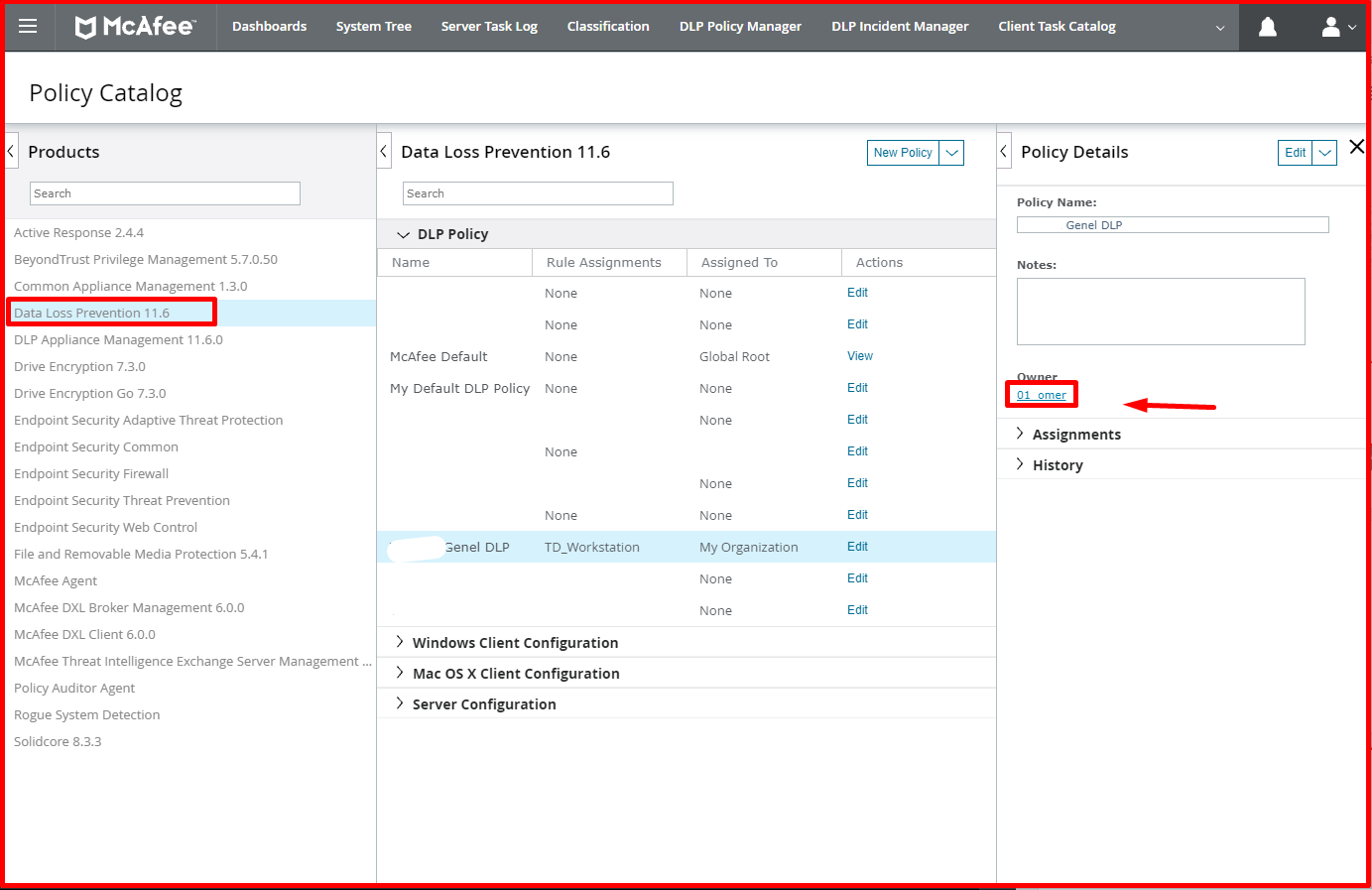This image displays a policy catalog for the software product McAfee (spelled as MAC-FE), focusing specifically on version 11.6 of its Data Loss Prevention (DLP) functionality. The catalog is organized into three columns: Products, Data Loss Prevention 11.6, and Policy Details.

The first column lists various McAfee products, including:
- Active Response 2.4.4
- BeyondTrust Privilege Management
- Common Appliance Management
- Data Loss Prevention (DLP)
- DLP Appliance Management
- Drive Encryption
- Drive Encryption Go
- Endpoint Security Adaptive Threat Protection
- Endpoint Security Common
- Endpoint Security Firewall
- Endpoint Security Threat Prevention
- Endpoint Security Web Control
- File and Removable Media Protection
- McAfee Agent
- McAfee DXL Broker Management
- McAfee DXL Client
- McAfee Threat Intelligence Exchange Server Management
- Policy Auditor Agent
- Rogue System Detection
- Solidcore Product

In the second column, the product Data Loss Prevention 11.6 is highlighted, indicating it is the focal point for this catalog entry. Information from the DLP policy is displayed, providing options to view configurations for the Windows client, the macOS X client, and the server. Of these, only the DLP policy itself is accessible.

The third column, Policy Details, includes specific information about the policy. The owner's name is listed as "010_M_ER" with spaces, and there are options to view assignments and the history of the policy details.

The entire layout suggests a well-organized catalog designed to provide clear and detailed information about various McAfee products, with a specific emphasis on Data Loss Prevention 11.6 and its associated policies.